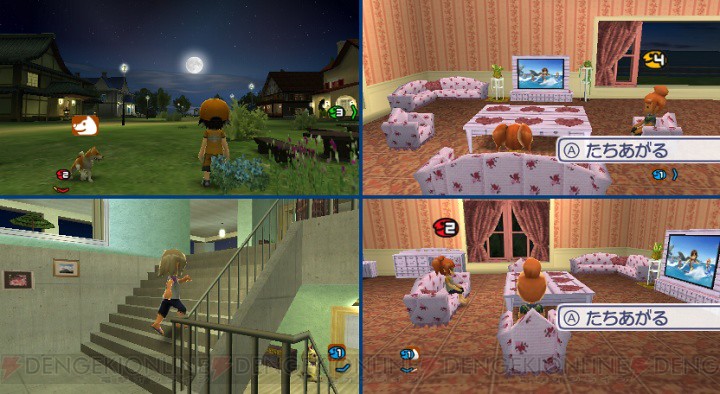This image is a collage of four interconnected pictures, divided by a blue vertical line in the middle and a blue horizontal line in the center, forming a quadrant layout.

**Top-Left Quadrant:** This appears to be a nocturnal scene possibly from a video game. It features a black sky dominated by a large, luminous moon casting its light on a range of mountains. Below, there is a street flanked by houses with some lights on, surrounded by green grass. In the foreground, a small cartoon character with his back facing the viewer is visible. He is wearing a brown baseball cap, a brown shirt, and shorts. Nearby, a picnic bench is adorned with plants. Additionally, there's a peculiar green-lit object near the house on the right and a small white horse figurine inside a box.

**Bottom-Left Quadrant:** This section shows an interior featuring a staircase. A figure clad in black shorts is ascending the stairs. The walls are painted green, and the staircase includes a landing with two framed pictures. 

**Top-Right Quadrant:** This depicts a room with a gold and orange patterned wallpaper on the upper section of the walls and green on the lower part. A large window reveals a nighttime view, accentuated with a yellow circle indicating the numeral '4'. Pink curtains are draped back, and the floor is carpeted in a pinkish burgundy hue. The room is furnished with pink furniture decorated with dark pink floral patterns, including a sofa, a chair, and an end table adorned with little red hearts. A television displaying floor plans is also present. A person is seen sitting on a love seat, while another figure bends over a piece of pink furniture with red flowers.

**Bottom-Right Quadrant:** Similar to the top-right quadrant, this image features the same pink floral furniture but at a different angle. The wallpaper includes a black circle with the numeral '2' unlike the yellow '4' in the upper room.

All the images cohesively illustrate a detailed and colorful setting, imbued with whimsical and serene elements.